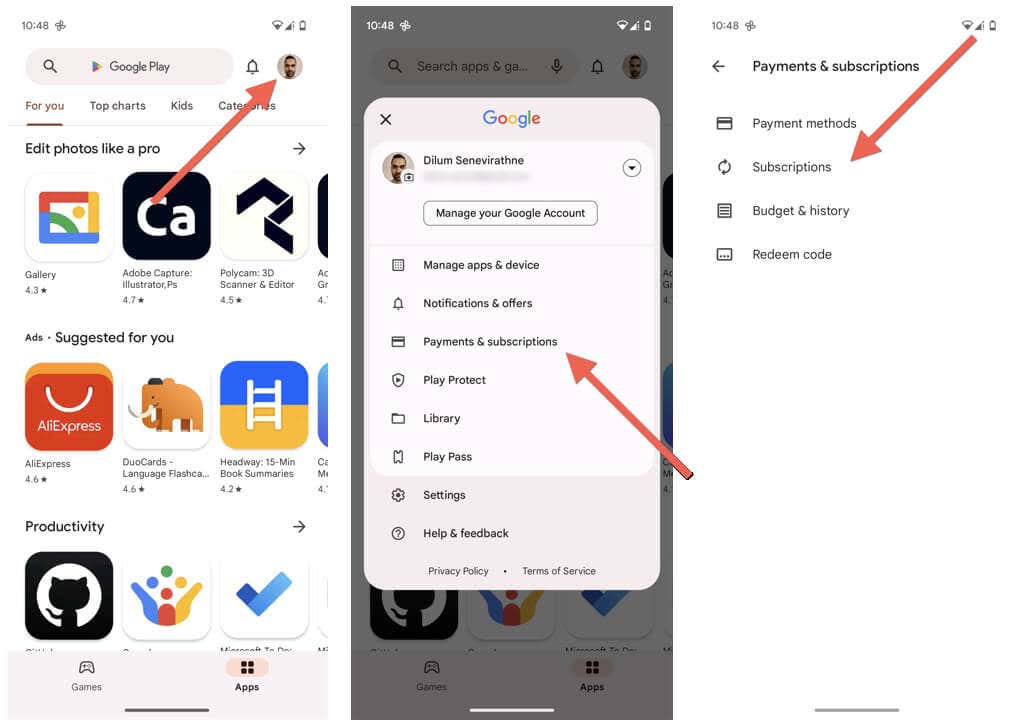The image displays three screenshots arranged side-by-side, each marked with a timestamp of 10:48. The first screen showcases the Google Play Store, highlighting the app Adobe Capture with a red arrow pointing towards the application's icon. Above the app icon, a caption reads "Edit photos like a pro," and the visible interface elements include options for galleries and other features.

The second screen depicts the user's Google account settings page. The page contains the user's name and the prompt to "Manage your Google account." Below this, various menu options are listed, such as "Manage apps and devices," "Notifications and offers," "Payments and subscriptions," "Play Protect library," "Play Pass," "Settings," and "Help and feedback." A red arrow specifically points to the "Payments and subscriptions" menu item, directing attention to it.

The third and final screen focuses on the "Payments and subscriptions" section of the Google account. Here, several options are presented, including "Payment methods," "Subscriptions," "Budget and history," and "Redeem code." A red arrow points toward the "Subscriptions" option, indicating its significance. This series of screenshots appears to illustrate the steps necessary to manage app subscriptions, with a possible intent of subscribing to Adobe Capture.